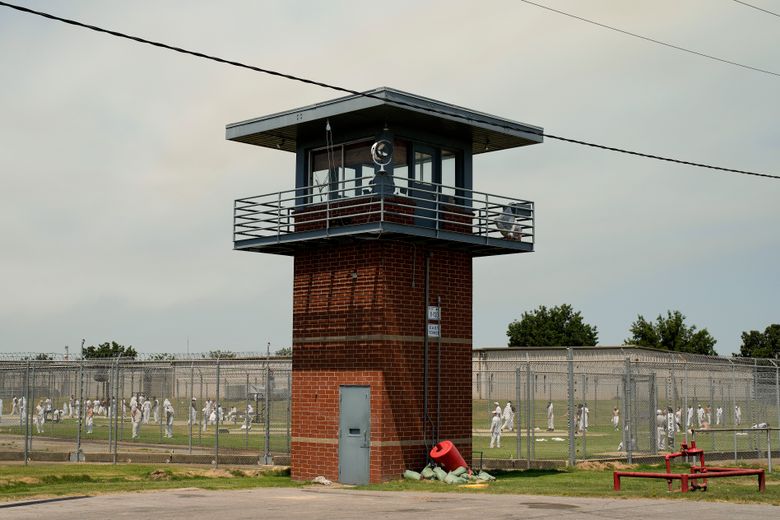The photograph depicts a prison yard dominated by a prominent red brick watchtower, approximately two stories high, featuring a single grey metal door at its base and grey railings around its upper level to prevent falls. The upper level of the tower has a roof and enclosed area where guards can oversee the yard, equipped with additional equipment, likely for enhanced surveillance. Surrounding the yard is a high fence topped with razor wire. Within the fenced area, around 50 inmates in white uniforms are seen walking and gathering on a grass field, basking in the sunlight. Power lines can be seen overhead, and patches of concrete intersperse the grassy area, contributing to the stark, secure atmosphere of the prison environment.